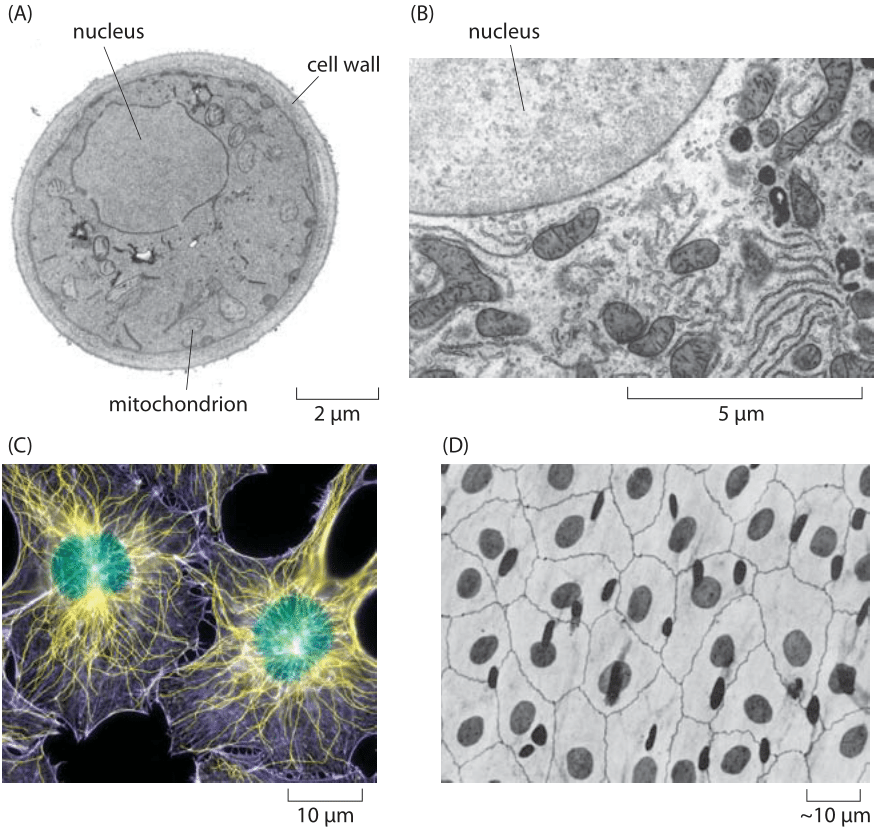The image comprises four scientific illustrations, each depicting the dimensions and structures of cellular nuclei using various microscopic techniques. 

In the upper left quadrant, labeled A, there's a black and white microscopy image of a single cell. Key structures such as the nucleus, mitochondria, and cell wall are clearly labeled, providing a context of the nuclear size with a scale of 2 micrometers.

To the right, in quadrant B, there's a closer, more detailed black and white view of the nucleus, showcasing the surrounding area including mitochondria and the Golgi apparatus. This image focuses on the nucleus with a measurement scale of 5 micrometers.

The bottom left quadrant, labeled C, features the only colored image. This fluorescent microscopy image displays a human fibroblast cell in vivid green, with the nucleus at the center lit up, surrounded by elements in hues of yellow and purple. This image provides a visual contrast and highlights the nucleus using colors to delineate different cellular components.

Finally, the bottom right quadrant, labeled D, shows another black and white image, but this time of a human epithelial sheet. The nuclei appear as dark ovals stained in silver, emphasizing the repetitive structure of many cells together. Both the images in the lower quadrants have a scale of 10 micrometers, unifying the depiction of cellular arrangements and their nuclei sizes.

Together, these illustrative sections present a comprehensive, detailed visualization of cellular nuclei across different cell types and microscopy techniques, each with precise measurements.